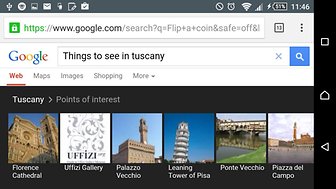Screenshot Description:

The screenshot depicts a mobile phone display with a dark blue border at the top, featuring various status icons including mail, WiFi signal, cellular signal strength, a 55% battery indicator, and the time displayed as 11:46. Below the status bar is an address bar showing the URL "https://www.google.com/search?q=flip+a+coin&safe=off8," which is secured as indicated by a green square containing a lock icon. Underneath the address bar, there is a Google search box displaying the query "things to see in Tuscany," flanked by the Google logo on the left and a magnifying glass (search icon) along with an 'X' (clear search) on the right. Below the search box, there are options labeled "Web," "Maps," "Images," "Shopping," and "More." The interface also includes a black section with six thumbnail images representing popular attractions in Tuscany. From left to right, these thumbnails are labeled as follows: Florence Cathedral, Uffizi Gallery, Palazzo Vecchio, Leaning Tower of Pisa, Ponte Vecchio, and Piazza del Campo.